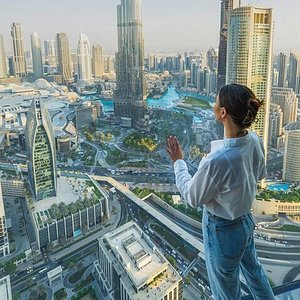The photograph depicts a woman standing indoors, looking out from a high vantage point through a window. She is positioned on the right side of the image, with her left hand touching the glass pane. The woman is dressed in a white long-sleeve button-down shirt and light blue denim jeans, with her brown hair neatly tied up in a bun at the back of her head. Although the image is small and somewhat blurry, it is clear that she is gazing out at a sprawling urban landscape below. The scene outside the window features a vast network of roads with numerous tiny cars navigating through them, flanked by an array of buildings and skyscrapers. Among these buildings, some have rooftops adorned with plants, giving the appearance of rooftop gardens. The cityscape also includes lush greenery with trees scattered throughout and various grassy areas. Further in the distance, there are watery expanses, possibly a river or a swimming pool, adding to the diverse elements that make up the bustling city view.